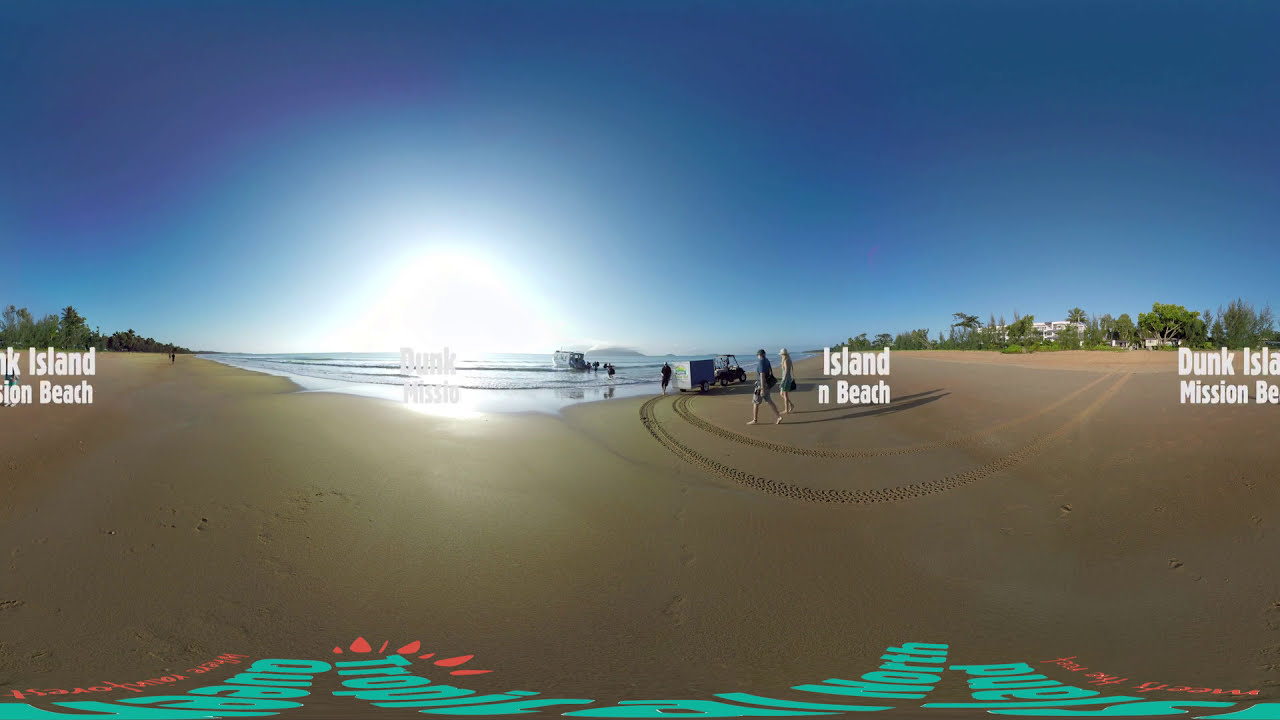A panoramic image captures a picturesque beach scene on Dunk Island, featuring a backdrop of deep blue skies and the shimmering ocean reflecting the sun's glare. The sandy beach, smooth with some footprints and indents, stretches out under a soft, beige hue. Prominently, signs displaying 'Dunk Island' and 'Mission Beach' in white font are scattered across the area, some partially cut off due to the panoramic view. In the background, several people walk along the shoreline while others enjoy the water under the diminishing daylight, suggesting the sun is setting. To the right and left of the central beach area, dense trees and bushes frame some visible buildings and a few houses. A dune buggy and a trailer, leaving imprints in the sand, are present, enhancing the lively summer day ambiance on this scenic island.